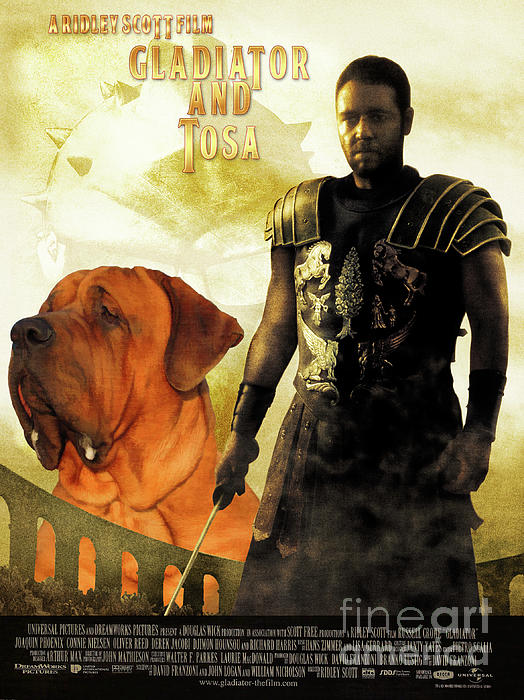This detailed movie poster features a golden to tan-orange background, with a faint outline of a man wearing a spiked hat. Central to the poster is a prominently displayed Gladiator, who is the same actor from the Gladiator movies. He is depicted with short hair, wearing intricate armor adorned with images of horses and a tree, and holding a sword. Surrounding him are architectural elements resembling old Roman aqueducts or possibly the Colosseum. Above him, the title reads "A Ridley Scott Film, Gladiator, Antosa." Towards the bottom, a brown dog with floppy ears and loose skin looks sideways to the left. There is also a Greek wall with fine print, likely listing the cast and crew, and a watermark saying "Fine Art America" in the bottom right corner.